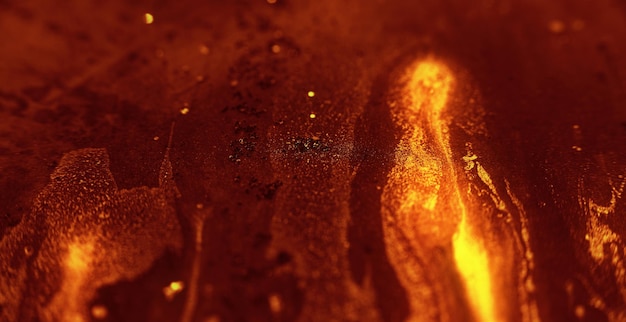This detailed, photorealistic image predominantly features a molten-like substance that closely resembles lava. The overall scene is dominated by hues of deep crimson red and burnt sienna, interspersed with vibrant swirls of orange and yellow. These colors create a dynamic and intense visual effect, mimicking the appearance of molten rock. The texture of the surface exhibits a bubbled and cracked pattern, with fissures revealing bright yellow beneath the darker red crust, adding to the illusion of molten material. Scattered sparks of yellow appear to dance across the image, contributing to the fiery atmosphere. The photograph portrays dripping formations that give a sense of substance flowing from a flat surface, enhancing its realistic magma-like quality. One prominent section to the right showcases a distinctive patch of what looks like true lava: a bright yellow core enveloped by gradients of orange to darker hues.